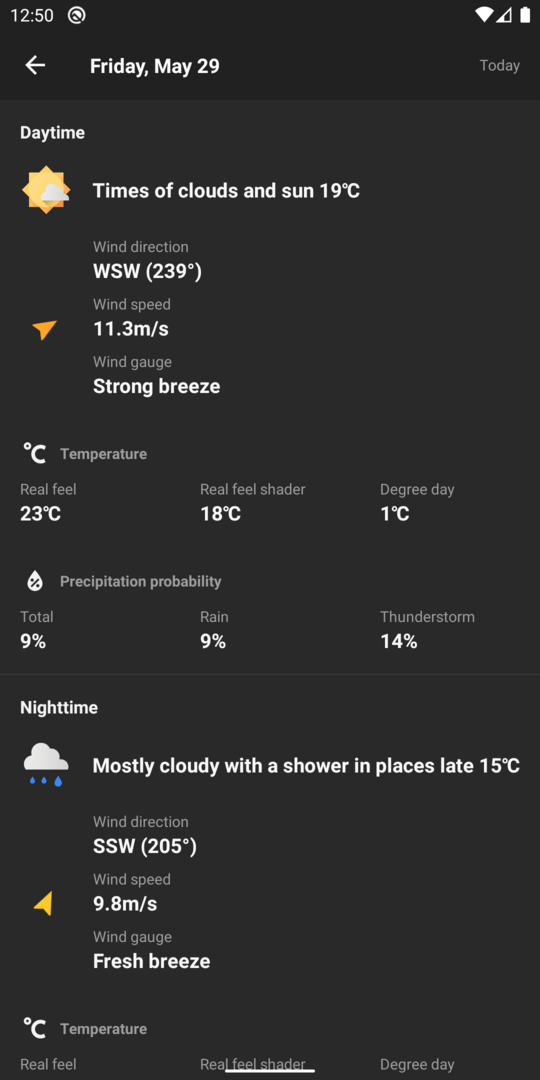**Image Description: Detailed Weather Forecast Display on a Cell Phone Screen**

The image captures a detailed weather forecast displayed on a cell phone screen, set against a black background. 

- **Top Left Corner:** The time is displayed as `12:50 PM`.
- **Top Right Corner:** Icons indicating battery life and Wi-Fi signal strength are visible.

**Header Section:**
- A white left arrow points back, suggesting navigation options.
- The date and time are displayed as `Friday, May 29, Daytime`.
  
**Daytime Forecast:**
- Two overlapping yellow squares and white clouds symbolize the weather conditions.
- The text beside the icon reads, "Times of Clouds and Sun, 19°C."
- Wind information: 
  - Direction: WSW (239°).
  - Speed: 11.3 M/S.
  - Wind description: "Strong Breeze."
- Temperature details:
  - Temperature: 19°C.
  - Real Feel: 23°C.
  - Real Feel in Shade: 18°C.
  - Degree Day: 1°C.
- Precipitation probability:
  - Total: 9%.
  - Rain: 9%.
  - Thunderstorm: 14%.
  
**Separator:**
- A thin gray line separates the daytime and nighttime forecasts.

**Nighttime Forecast:**
- The header indicates "Nighttime."
- An icon of a cloud with three blue raindrops represents the weather.
- Text reads, "Mostly Cloudy with a Shower in Places Late, 15°C."
- Wind information:
  - Direction: SSW (205°).
  - Speed: 9.8 M/S.
  - Wind description: "Fresh Breeze."
- Additional temperature details (though not fully shown in this summary):
  - Real Feel: 
  - Real Feel in Shade: 
  - Degree Day:

The image provides comprehensive weather information, presented in a clear and organized manner, for both daytime and nighttime periods.